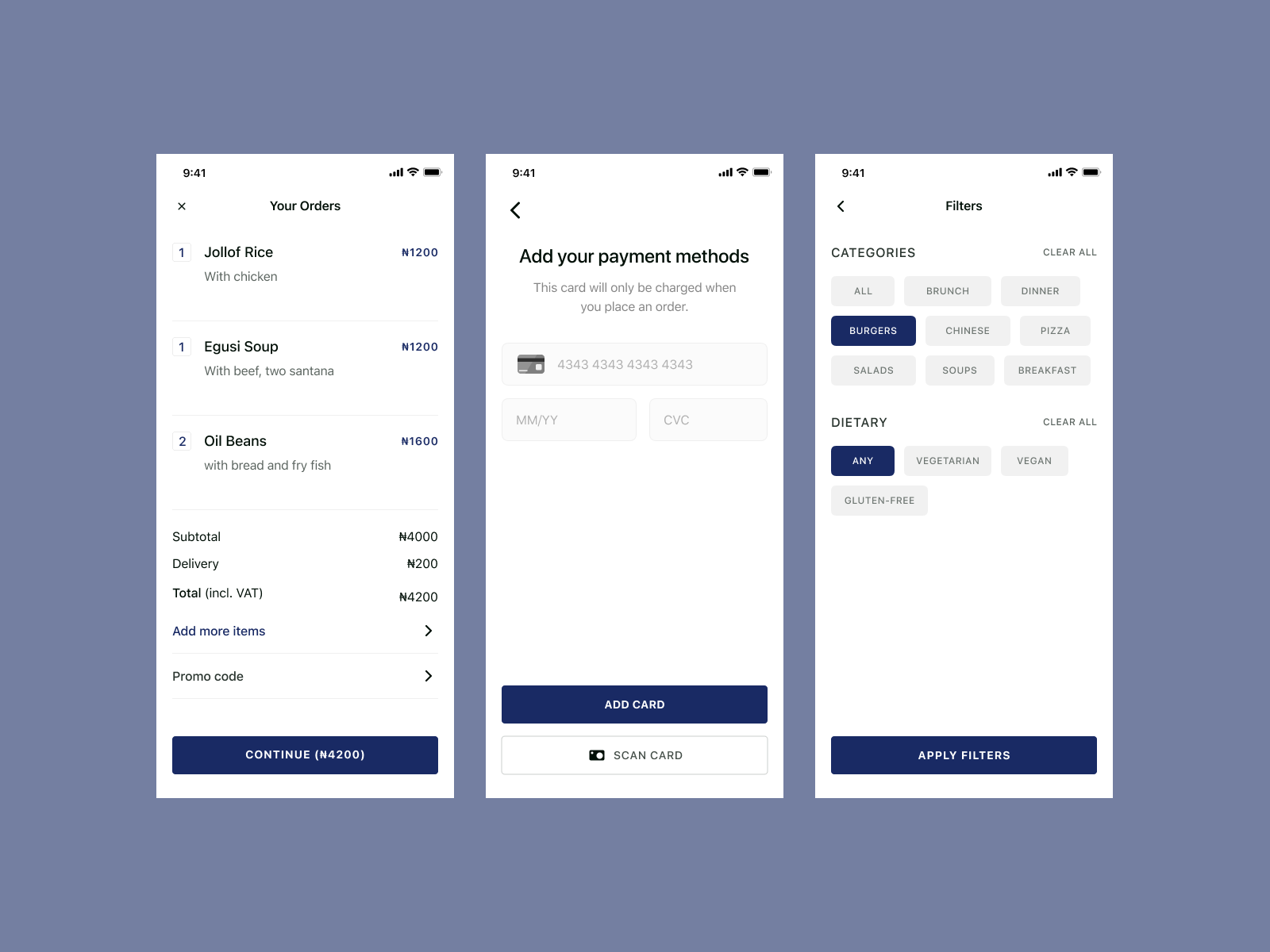In this composite photograph, three distinct screenshots are displayed against a gradient background transitioning from white to periwinkle blue. Each screenshot is uniformly timestamped at 9:41 and offers a detailed portrayal of different stages of a food delivery app's interface.

The first screenshot on a white background reveals the "Your Orders" page, presenting a comprehensive summary of the order details. The top bar indicates a strong carrier signal, active Wi-Fi connection, and a nearly full battery. An 'X' button in the top left corner allows users to exit. The order list includes:
- One Jollof rice with chicken priced at ₦1200
- One Egusi soup with beef at ₦1200
- Two Santana oil beans with bread and fried fish costing ₦1600
The subtotal adds up to ₦4000, with an additional delivery fee of ₦200 bringing the total, inclusive of VAT, to ₦4200. This page also offers an option to add more items and apply a promo code.

The middle screenshot focuses on the "Add Your Payment Method" section, offering users the choice to either add a new card or scan an existing one for payment processing.

The third screenshot, likely displaying the "Applying Filters" section, allows users to refine their search or order preferences to enhance their user experience.

Overall, this collage of screenshots provides an insightful glimpse into the functionalities and user interface of the food delivery application.